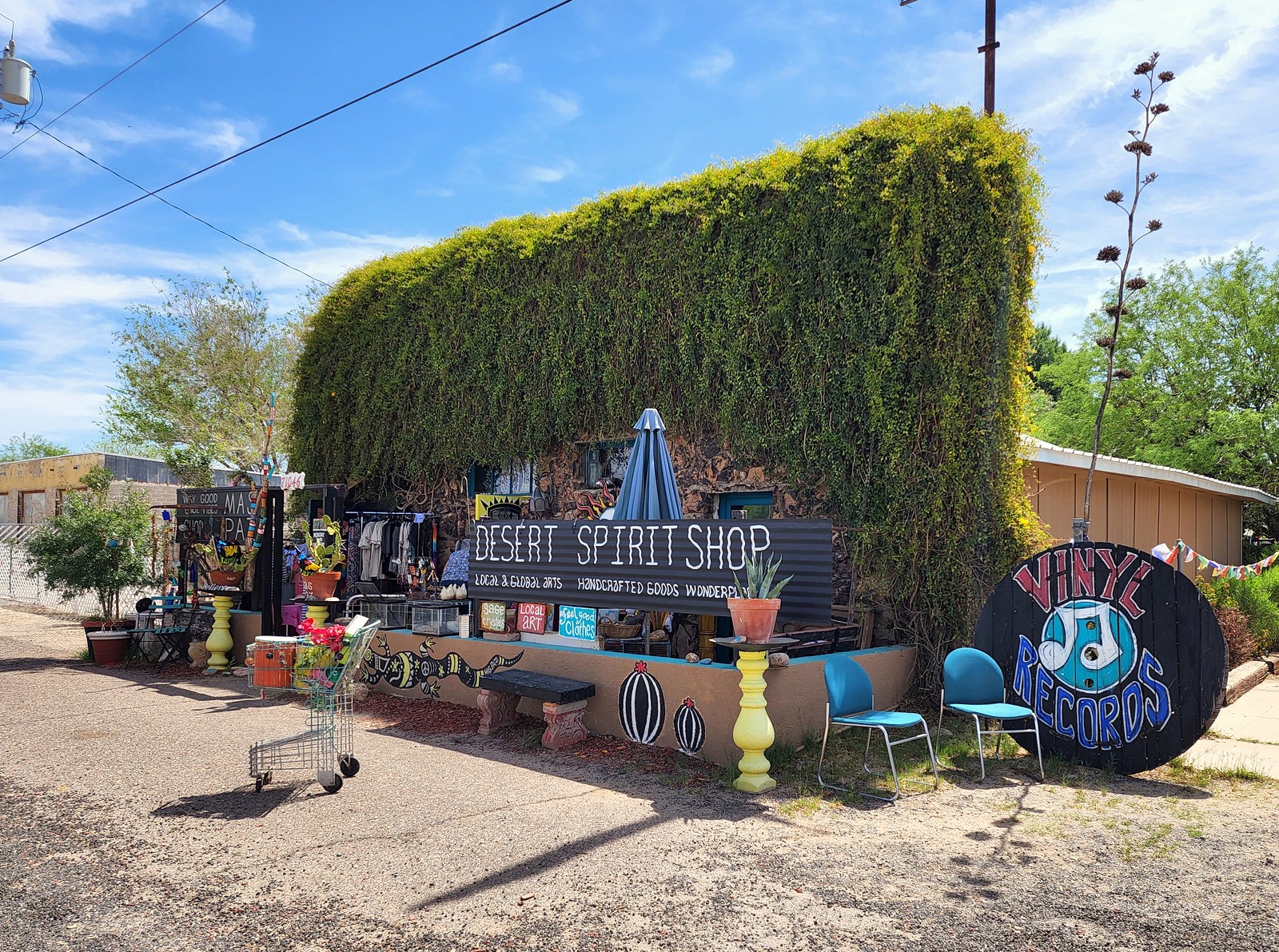The image depicts a unique and eclectic storefront called the Desert Spirit Shop, situated in the center of the frame against a backdrop of a bright blue sky with feathery white clouds and intersected by a telephone line at the top. The shop itself resembles a small brown shack with a white roof, partially obscured by tall, draping trees and possibly ivy or similar vegetation that almost hides the windows, giving the shop a charming, overgrown look. The ground in front is primarily gravelly with small rocks, and there are elements of both paved and unfinished surfaces.

The sign for the shop is metal, prominently displaying "Desert Spirit Shop" in white capital letters. Below it, in smaller text, it advertises "handcrafted goods" and another indistinct phrase. A smaller circular wooden sign to the right reads "vinyl records," with "vinyl" in red, "records" in blue, and a musical note in between, clearly painted on.

In front of the shop, there's an assortment of eclectic items: several statues that double as stands, each holding potted plants with sharp, pointy green leaves; various trinkets; colorful vases; and blue chairs. There is also a grocery cart visible, suggesting a whimsical and eclectic mix of items typical of a vintage thrift store crossed with an arts and crafts shop. To the left, another business can be faintly seen, adding to the charm and residential feel of the setting. This image captures the adventurous and bohemian spirit of the Desert Spirit Shop, promising a fun and intriguing experience inside.